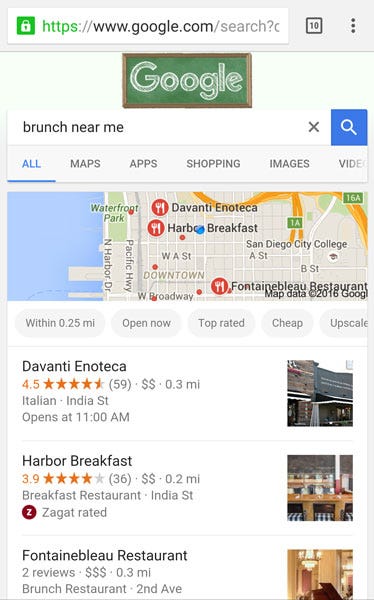This image appears to be a screenshot from a mobile device, either a phone or a tablet. At the top of the screen, the URL "http://www.google.com" is visible, along with a small square box displaying the number "10," likely indicating the number of open browser tabs. Below the URL bar, there's a prominent Google logo displayed on a green chalkboard with the word "Google" written in white chalk.

In the search query field, the phrase "brunch near me" is entered, accompanied by a blue "Search" button. Beneath the search bar, navigation tabs labeled "All," "Maps," "Apps," "Shopping," "Images," and "Videos" are present, with the "All" tab currently highlighted.

The search results include a map highlighting key locations in the area, such as San Diego City College, Downtown, Pacific Highway, Waterfront Park, Devanti Enoteca, and Harbor Breakfast. The map provides detailed information about nearby brunch spots:

1. **Devanti Enoteca** - An Italian restaurant located 0.3 miles away from the user, rated 4.5 stars from 59 reviews, situated on India Street, and opens at 11 a.m.

2. **Harbor Breakfast** - A breakfast restaurant situated 0.2 miles away, with a rating of 3.9 stars from 36 reviews, located on India Street and recognized by Zagat.

3. **Fountain Blue Restaurant** - A brunch restaurant located on Second Avenue, 0.3 miles away. It has two reviews but does not display a star rating.

This detailed breakdown offers a comprehensive overview of the search interface and the specific brunch options available near the user's location.